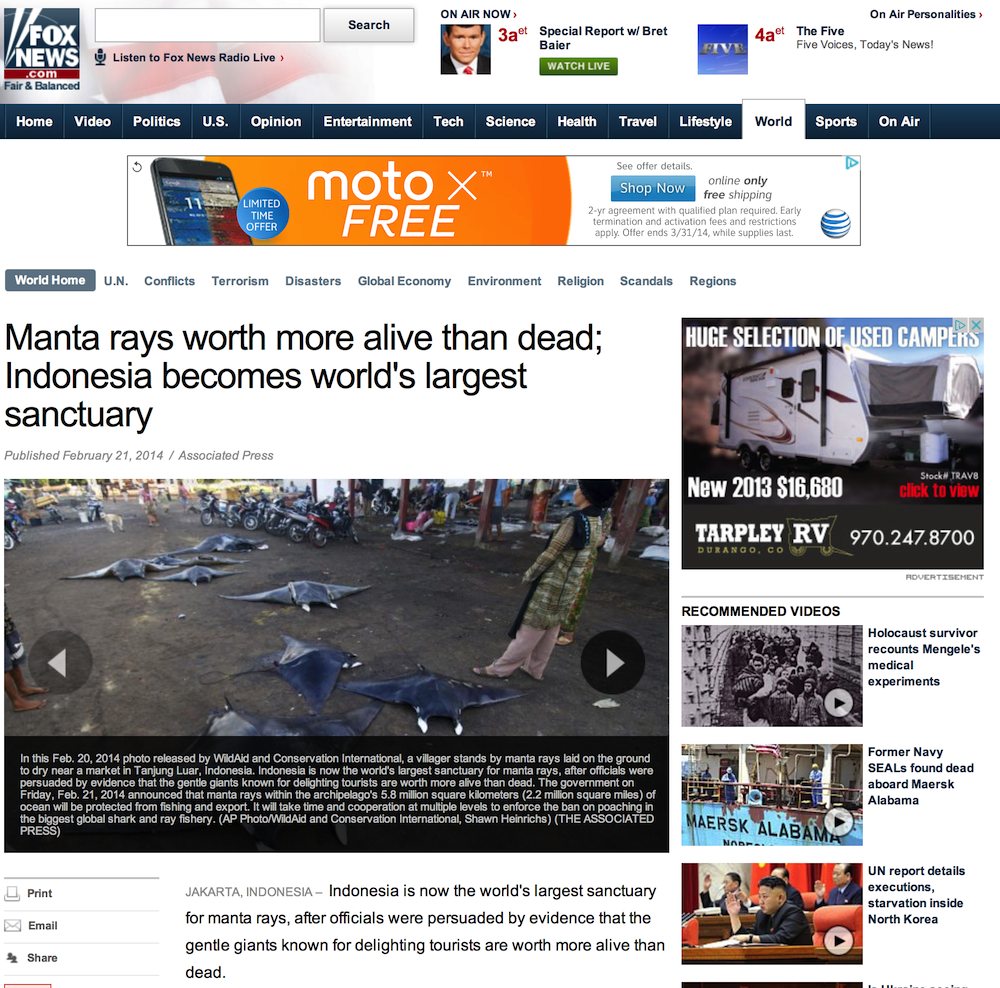Detailed Caption for the foxnews.com Image:

The image captures the homepage of the foxnews.com website. In the top left corner, adjacent to the Fox News logo, there is a search bar for easy navigation. Beside the search bar, there is an option to listen to Fox News Radio Live via a small link. Additionally, there is an "On Air Now" link highlighting a special report with Brett Baier, allowing users to watch live coverage.

Below this header, a blue navigation banner displays a series of primary categories including Home, Video, Politics, US, Opinion, Entertainment, Tech, Science, Health, Travel, Lifestyle, World, Sports, and On Air, with 'World' presently selected. 

Under the 'World' section, several subheadings are available: World Home, UN, Conflicts, Terrorism, Disasters, Global Economy, Environment, Religion, Scandals, and Regions. The 'World Home' subheading is currently active.

Dominating the main content area of the page is a headline story about manta rays. The article discusses Indonesia's establishment of the world's largest sanctuary for manta rays, emphasizing their higher value alive than dead. This main story is accompanied by an image of manta rays and a brief explanatory paragraph.

On the right side of the page, there is a prominent advertisement for a wide selection of used camper vans. Beneath the ad, a series of recommended videos are listed. The highlighted videos cover topics including the Holocaust, the discovery of dead former Navy SEALs, and issues pertaining to North Korea.